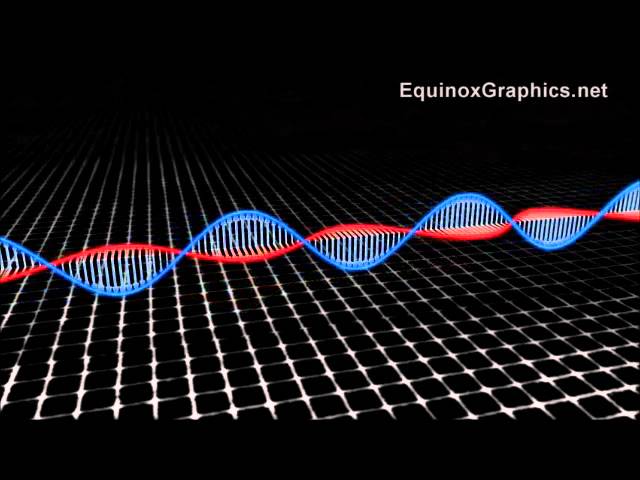The advertisement from EquinoxGraphics.net features a striking and minimalist design. Positioned against a black background, there is a white grid pattern on the lower section that resembles a floor or base, which fades into the background. The focal point of the image is a vivid representation of a DNA strand, depicted with undulating red and blue lines weaving through the center of the scene. Connecting these lines are numerous white bars, mimicking the helical ladder structure typical of DNA. The imagery extends from the left to the right side, invoking a sense of continuity and movement. In the top right corner, the website "EquinoxGraphics.net" is prominently displayed in white text, adding branding to the sleek and scientific visual.